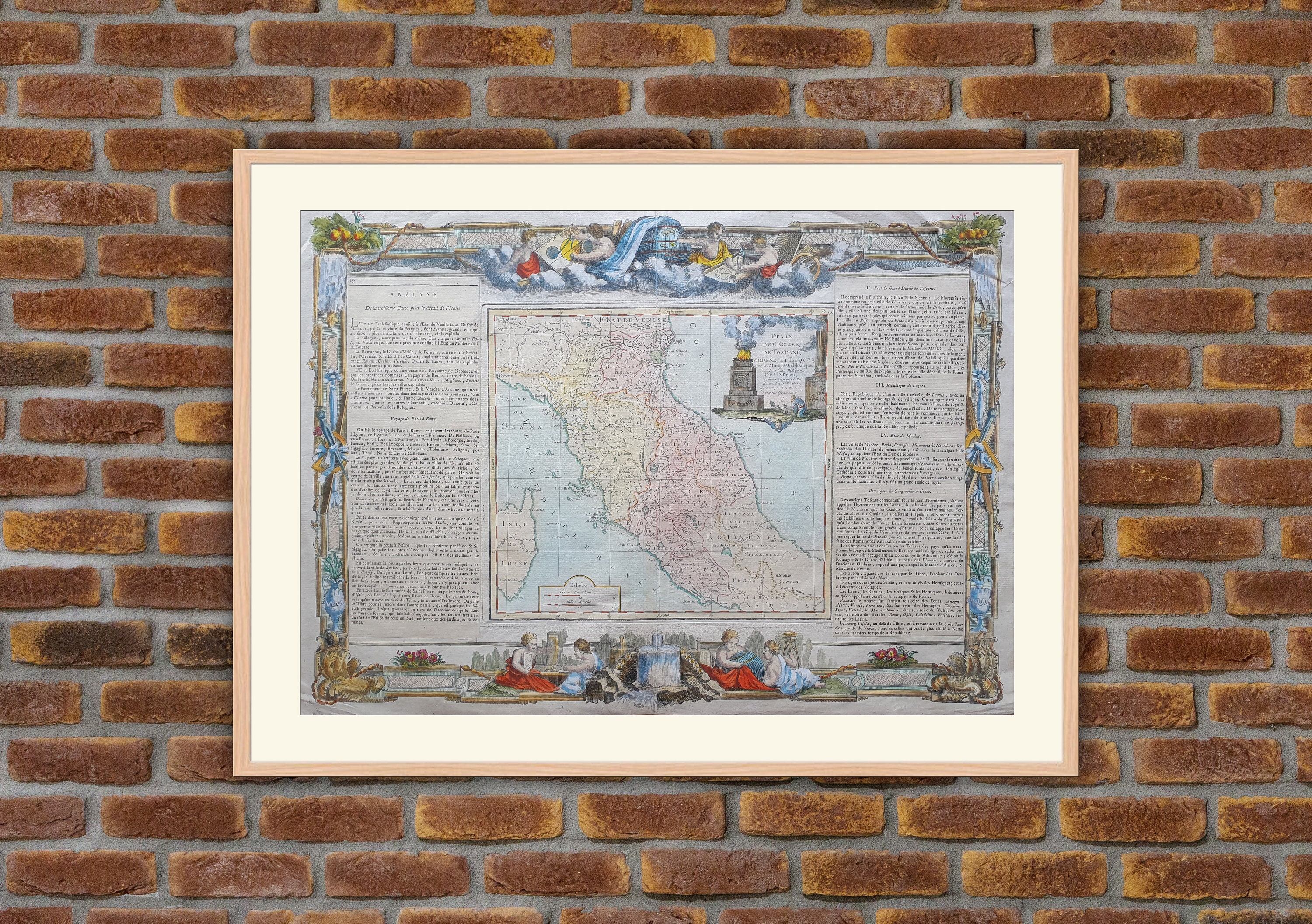The image depicts a framed map hanging on a light reddish-brown terracotta brick wall with gray cement. The map is encased in a light brown wooden frame, which is surrounded by a white border. The central focus of the picture is an ancient-style map that appears to depict Italy, displaying a peninsula with light blue seas on both sides and accented with sections in light pink and bright colors. Flanking the map are columns of text on both the left and right sides, though the exact details of the text are not legible. Encircling the map is a decorative border featuring intricate designs of various kinds of vegetation, fruits, and children or cherubic angels engaged in playful activities, giving the piece a royal and slightly religious aura. The lower part of the map hints at a cityscape, enhancing the detailed and historical ambiance of the artwork.